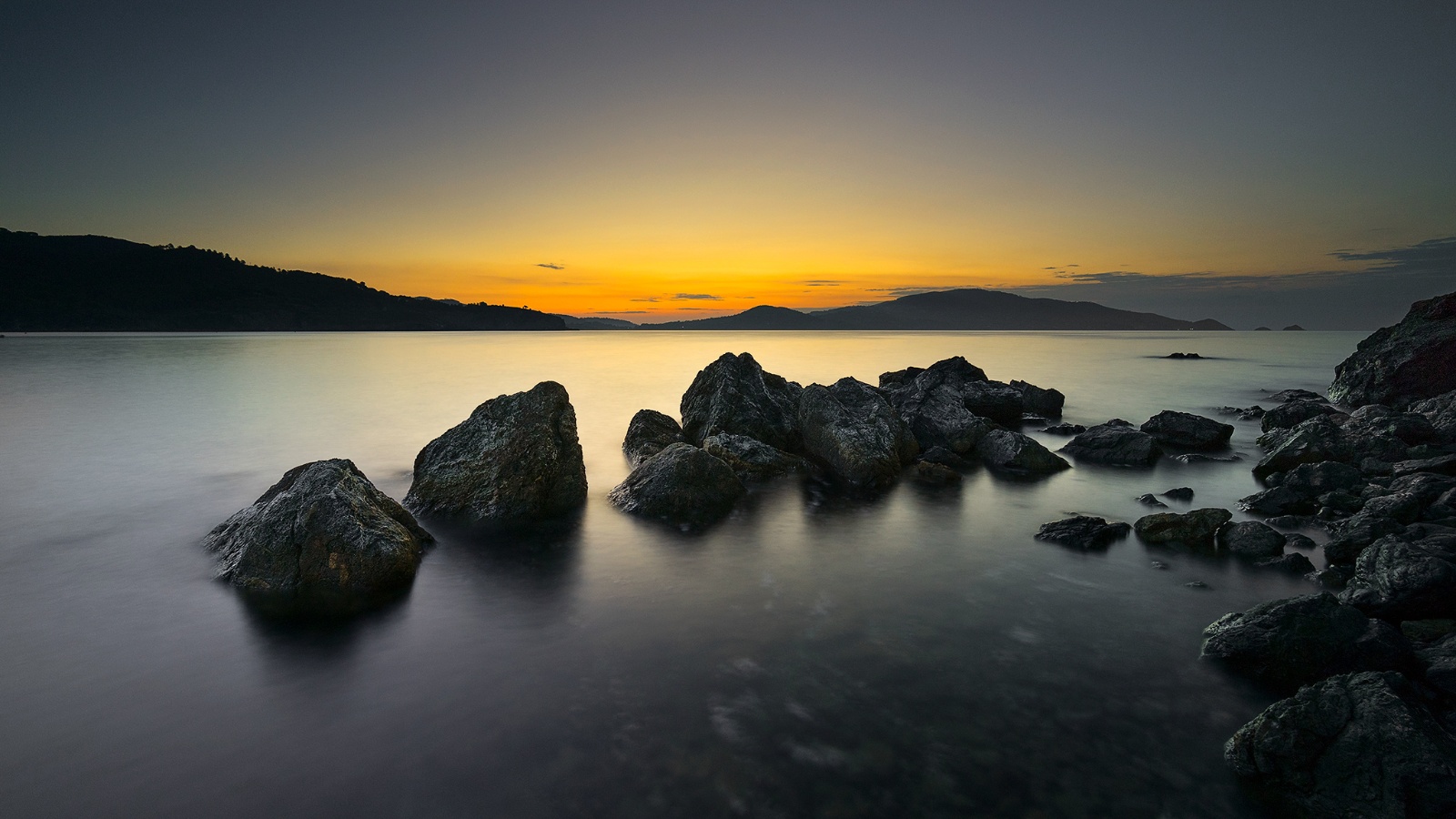The image depicts a tranquil aquatic scene during either sunset or sunrise, framed in a horizontal rectangle. The sky is transitioning through a palette of deep blue to reddish-orange hues near the horizon, suggesting the imminent arrival of the sun. The glow of the sky reflects subtly on the still, flat body of water, creating a velvety, smooth appearance. Along the left side of the image, dark gray, mountainous hills subtly silhouette against the sky. In the foreground, large, chunky rocks and boulders, varying in size, jut out from both the shoreline and the water itself, predominantly on the right-hand side. The entire scene is accentuated by the serene and reflective nature of the water, with a few wispy clouds adding texture to the sky. Despite the low lighting, the overall atmosphere is calm and picturesque, capturing a perfect moment of dawn or dusk.